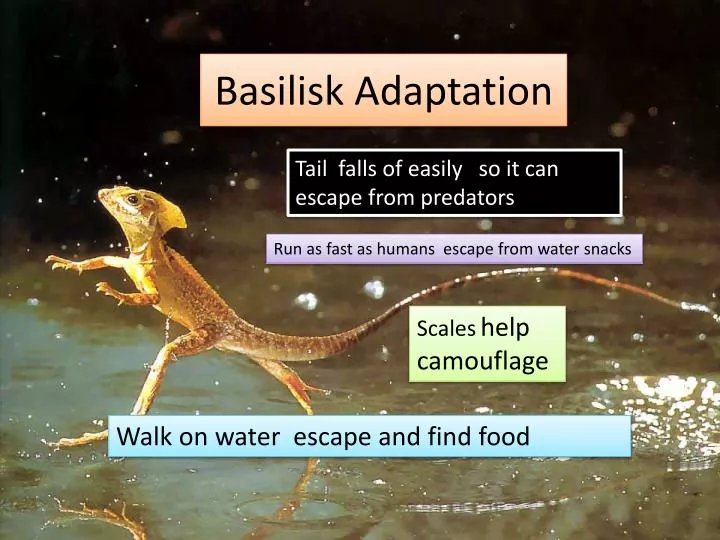The image is a slide from a PowerPoint presentation or a learning visual aid about the Basilisk lizard, commonly known as the "Jesus lizard" for its ability to run on water. The background photo features the light brown, spotted Basilisk in mid-stride, running on its hind legs across a body of water, with water splashing around its feet. The lizard's long tail extends out towards the right, and it has a distinctive pointy crest on its head reminiscent of a shark fin. 

At the top of the slide, a headline in a peach-colored box reads "Basilisk Adaptation." Below that, a series of text boxes provide detailed information about the lizard's unique traits:
1. A black box with white letters states, "Tail falls off easily so it can escape from predators," though "off" is misspelled as "of."
2. A light purple box claims, "Run as fast as humans, escape from water snacks."
3. A green box under the lizard’s tail notes, "Scales help camouflage."
4. Finally, a light blue box at the bottom concludes with, "Walk on water, escape, and find food."

The overall layout and the detailed presentation suggest it might be a student project designed to highlight the remarkable adaptations of the Basilisk lizard.